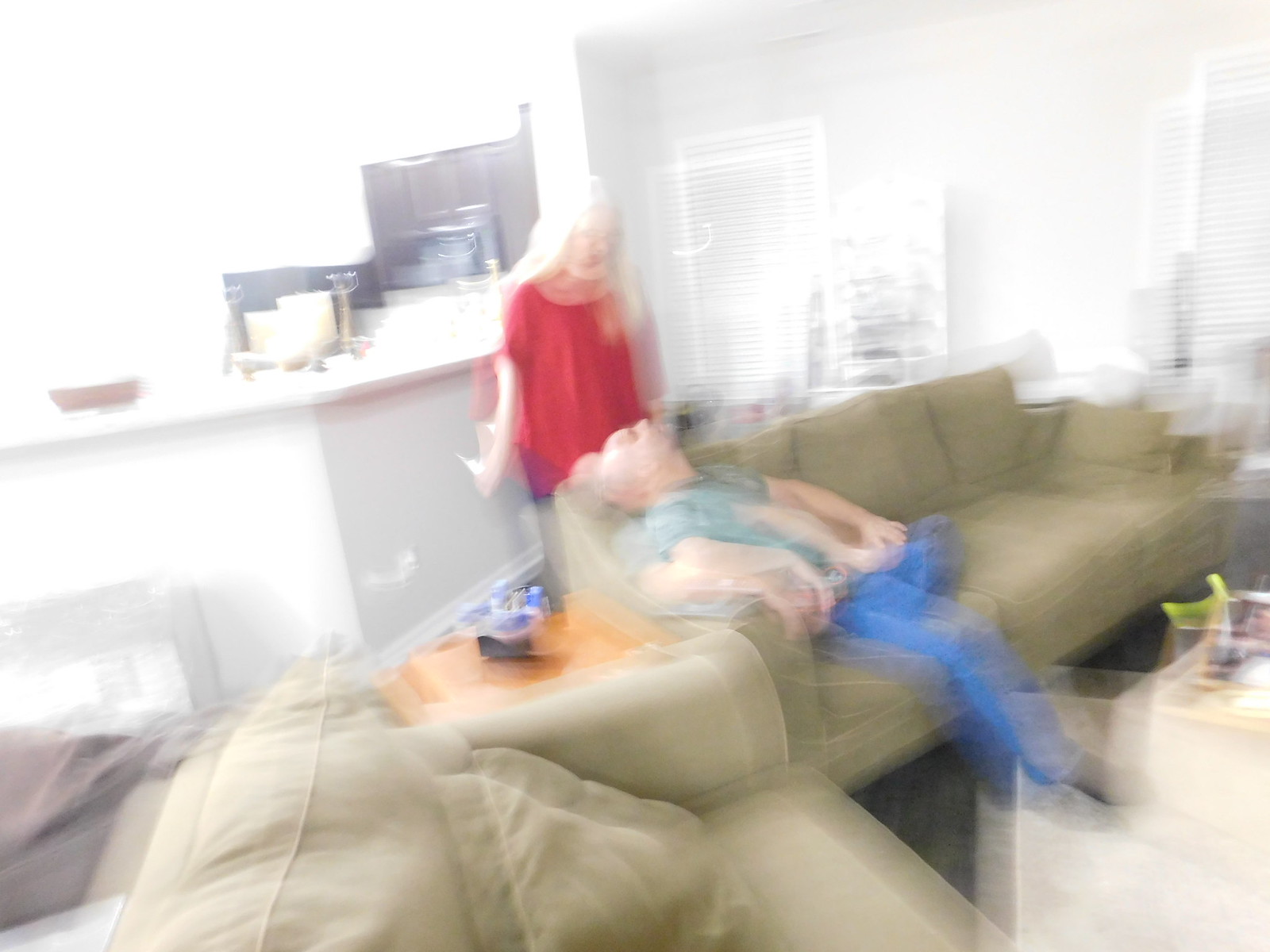In this very blurry and out-of-focus photograph, the scene is set in what appears to be a living room or sitting room with predominantly white walls and decor. The background features a white counter on the left side, adorned with several brown and black objects. On the right side, two white-trimmed windows with white blinds allow light to filter into the room, further brightening the predominantly white background.

The main focus of the photograph is two olive green sofas arranged at an angle to each other. Seated on one of these sofas is a man with white skin, dressed in a green shirt and blue pants. He is gazing upward. Directly behind the man's head stands a woman with white skin and long, light hair, wearing a red shirt.

Central to the two sofas is a square wooden table, adding a touch of warmth to the otherwise neutral color palette of the room.